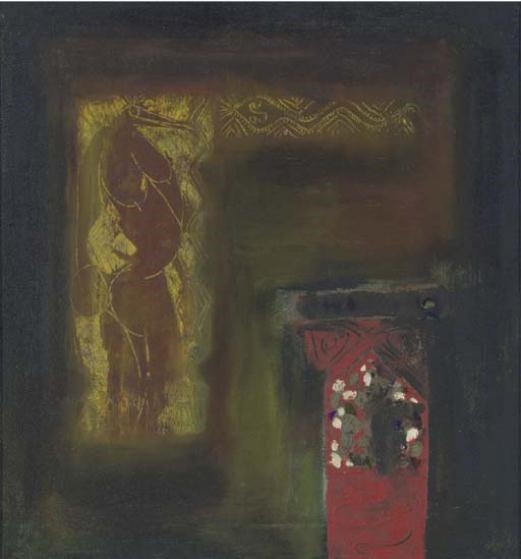This abstract painting presents a dark and complex canvas featuring predominantly blacks, dark browns, olive greens, and hints of yellow and gray. Dominating the upper left-hand portion is an upside-down L-shaped form with a dark brown background, highlighted by lighter yellow brushstrokes and green accents along its edges. The central area and surrounding portions are marked by a mix of blurry, unfinished strokes of green and olive green, blending into the backdrop. On the lower right-hand side, a prominent red rectangular shape draws attention, adorned with patches of dark gray, medium gray, white, and two purple dots. The painting overall exudes a dark, moody atmosphere with a mix of discernible and abstract elements, making it intriguing and hard to decipher.